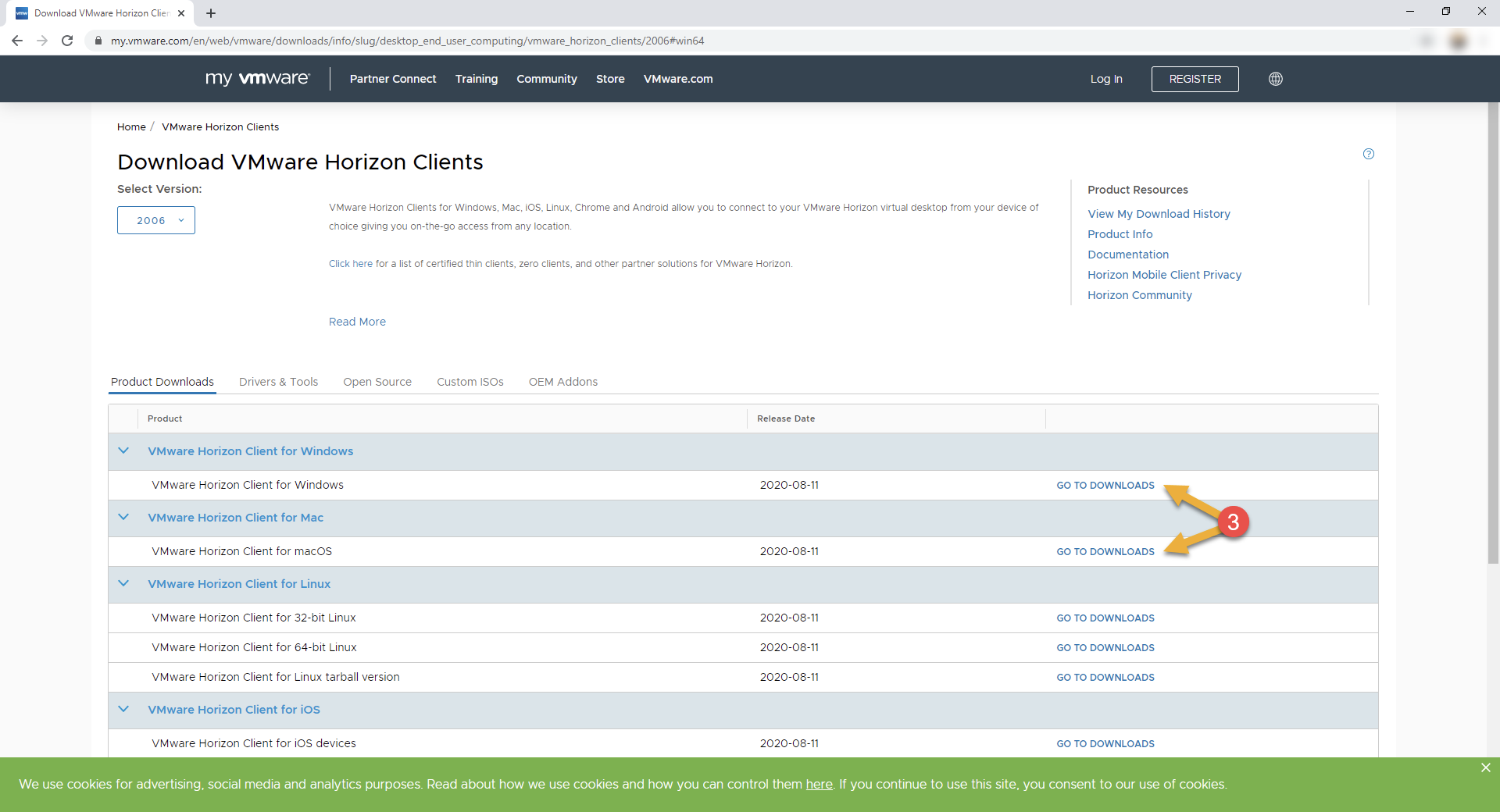This image showcases the User Interface (UI) of the "My VMware" portal. At the top, there's a striking blue banner displaying several navigation options: "Partner Connect," "Training," "Community," "Store," and "VMware.com," with options to "Log In" or "Register."

Beneath the blue banner, the background shifts to a clean white, highlighting primary options such as "Home," "VMware Horizon Clients," and "Download VMware Horizon Clients." A dropdown menu labeled "Select a Version" is visible, featuring "2006" in the blue box.

The main section details the "VMware Horizon Clients," which are available for various operating systems, including Windows, Mac, iOS, Linux, Chrome, and Android. These clients enable users to seamlessly connect to their VMware Horizon virtual desktop from any device, providing flexible access from any location. There's an actionable link that reads "Click here for a list of certified clients, zero clients, and other partner solutions for VM Horizon," followed by a "Read More" link in blue text. The "Product Downloads" link is prominently underlined in blue.

Noticeably, two options are highlighted with a round red circle containing the number three, accompanied by mustard-colored arrows pointing to the right. This emphasizes the "VMware Horizon Client for Windows" and the "VMware Horizon Client for Mac OS."

At the bottom, a green box states, "We Use Cookies for Advertising, Social Media, and Analytic Purposes." It encourages users to "Read about how we use our cookies and how you can control them here." Continued use of the site implies consent to the use of cookies.